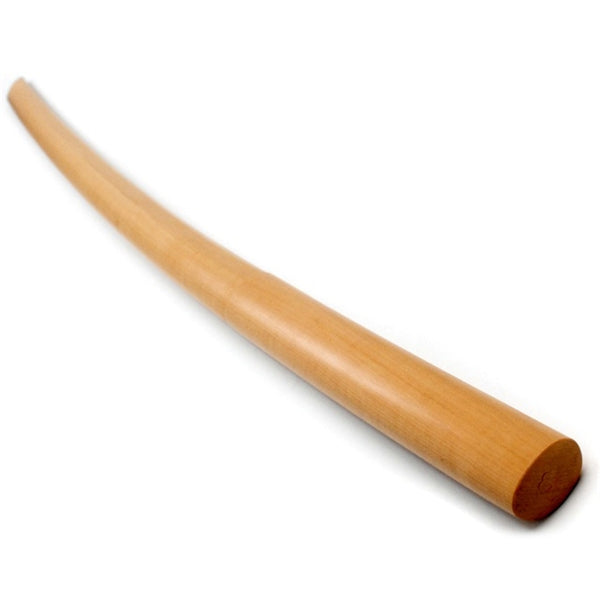The image depicts a highly polished, honey-colored wooden dowel resting on a white background. The dowel, reminiscent of an old-fashioned baseball bat or a training wooden sword, is circular in shape and tapers from a thicker bottom right portion to a narrower, curved upper left end. The wood's striations run along its length, and the object casts a subtle shadow that branches out predominantly downward, with additional shadowing visible on either side, especially towards the right back end. The dowel's smooth surface gleams, accentuating its finely crafted form.